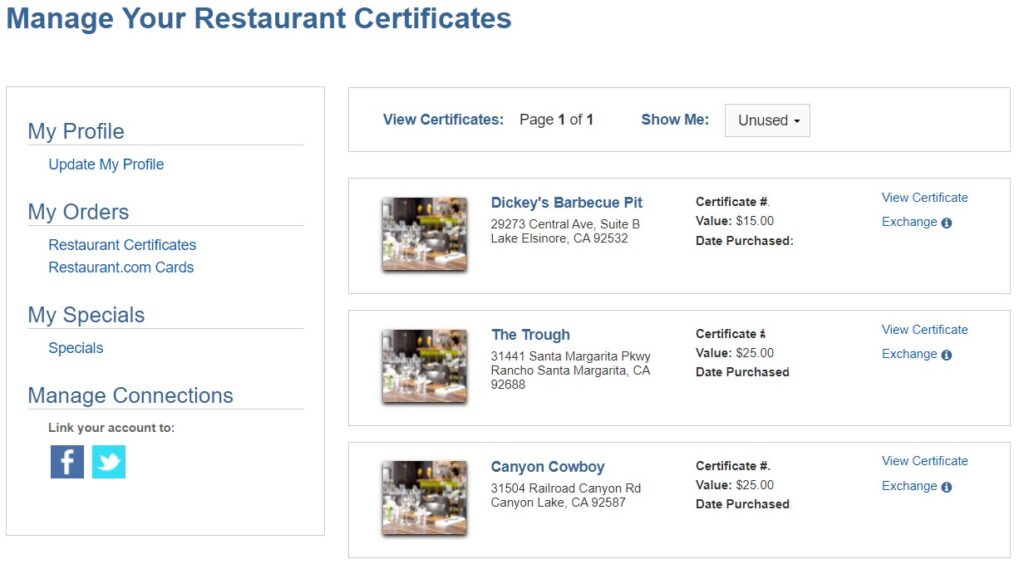The image displays a detailed interface of a restaurant management platform. The interface includes various sections such as "Manage Your Restaurant Certificates," "My Profile," "Update My Profile," "My Orders," and "Restaurant Certificates." Additional features include options for managing "Restaurant.com Cards," accessing "My Specials," "Manage Collections," and linking accounts to social media platforms like Facebook and Twitter.

Highlighted certificates include:
1. **Dickie's BBQ Pits**
   - Address: 29273 Central Avenue, Suite B, Lake Elsinore, California 92532
   - Certificate Value: $15
   - Functions: View Certificate, Exchange
   - Additional Info: Unused

2. **Santa Margarita**
   - Location: 31441 Santa Margarita Pkwy, Rancho Santa Margarita, California 92688
   - Certificate Value: $25
   - Functions: View Certificate
   - Purchased: Second Withdrawal

3. **Canyon Cowboy**
   - Address: 31504 Railroad Canyon Road, Canyon Lake, California 92587
   - Certificate Value: $25
   - Functions: View Certificate, Exchange
   - Additional Info: Date Purchased

Each section and certificate detail is accessible, allowing users to manage and exchange certificates seamlessly.